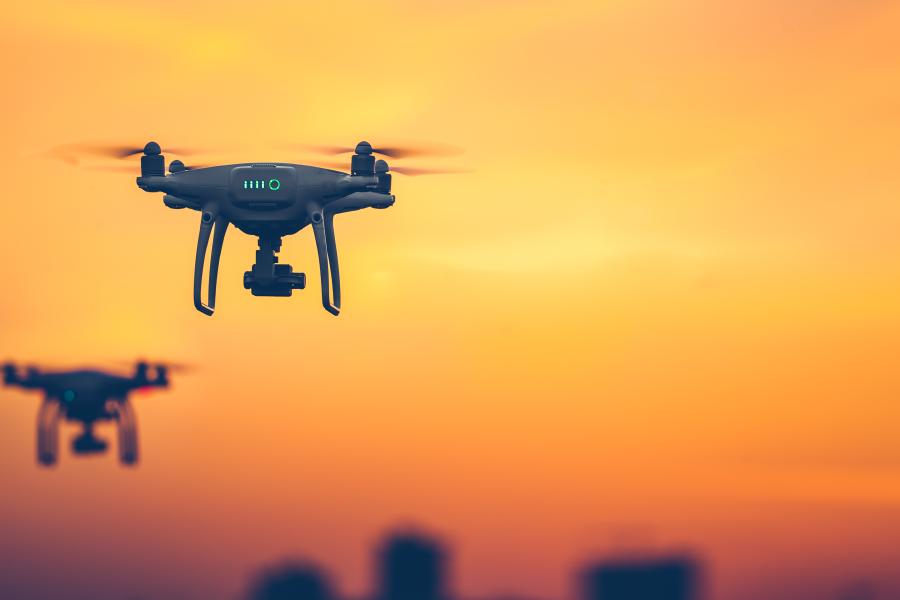In this photograph, two commercially-made drones hover against a vibrant sunset sky, which transitions from bright orange at the top to darker, reddish hues near the bottom. The sky’s gradient frames the image, adding depth and warmth. The foreground features a detailed, sharply-focused gray drone, likely a high-end DJI model. This drone has a sleek unibody design with four propellers in motion, creating a blur effect. Mounted underneath is a large camera, and a green LED power indicator on its side suggests it is fully powered.

In the background, a second drone, identical to the first but slightly smaller due to its distance, is partially obscured by a blurred depth of field. The bottom portion of the image reveals the hazy silhouettes of a cityscape with the tops of a few buildings just visible, adding a touch of urban intrigue to the scene. The overall composition balances the sophisticated technology of the drones with the natural beauty of the sunset.